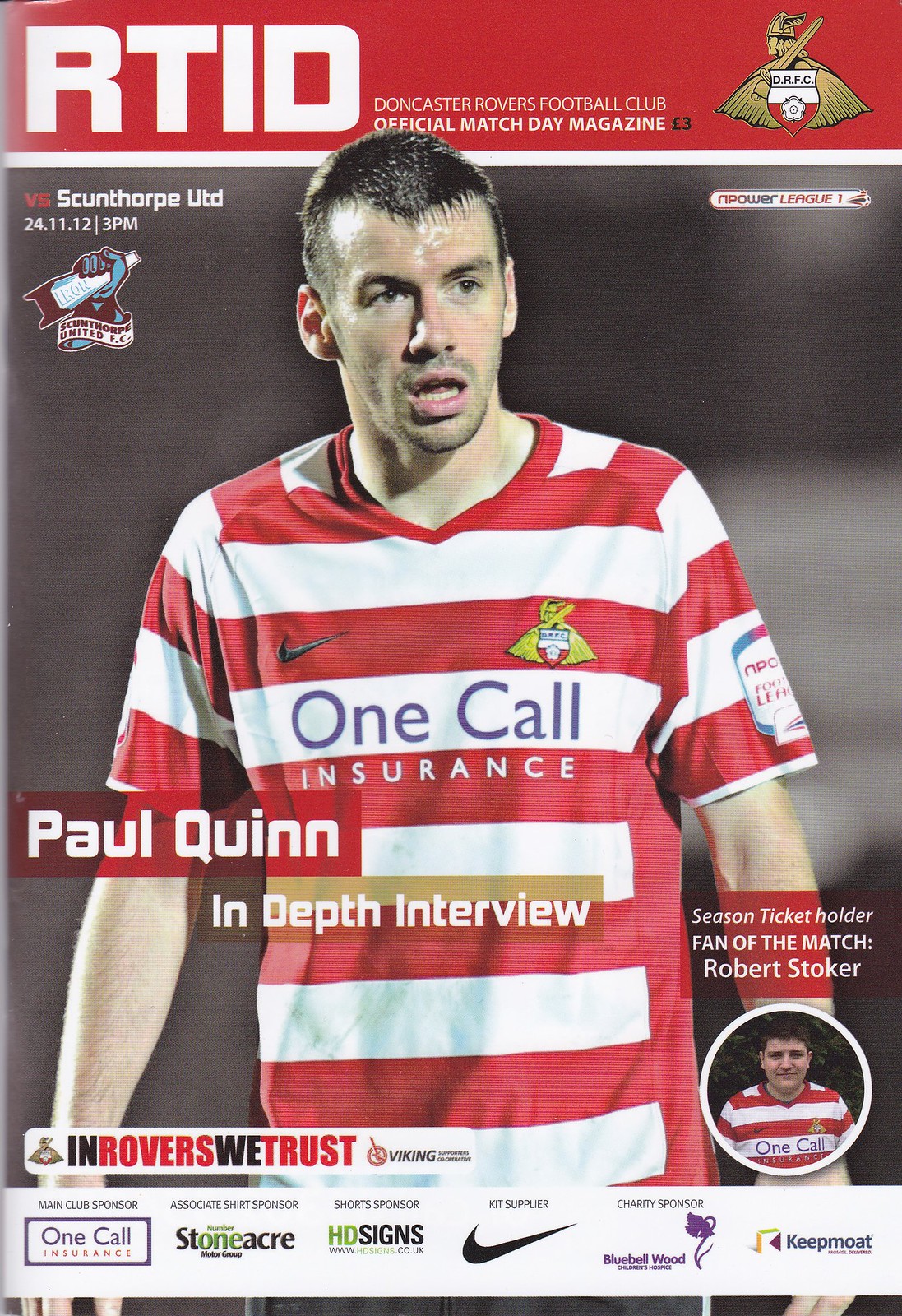The image is the cover of an official matchday magazine for Doncaster Rovers Football Club. At the top, a red horizontal bar features prominent white text that reads, "R.T.I.D. Doncaster Rovers Football Club Official Match Day Magazine." Next to this, in smaller black font, is the price, "£3." The cover prominently displays a young male soccer player wearing a red and white striped jersey with the "Nike" logo and the "One Call Insurance" branding, where "One Call" is in purple and "Insurance" in white. To the right of the player in an opaque red box with white text, it says, "Paul Quinn." Below this, in an opaque gold box with white text, it says, "In-Depth Interview." The player's background is gray. Additionally, there are various other texts and logos: "Scunthorpe Utd 24 11 12 3 p.m," "Season Ticket Holder Fan of the Match Robert Stoker," and "Empower League." The bottom section of the cover features several company logos and mentions sponsors such as One Call Insurance, Stoneacre, and HD Signs. The club's warrior logo holding a sword is also present, emphasizing the competitive spirit of the featured match against Scunthorpe United FC.